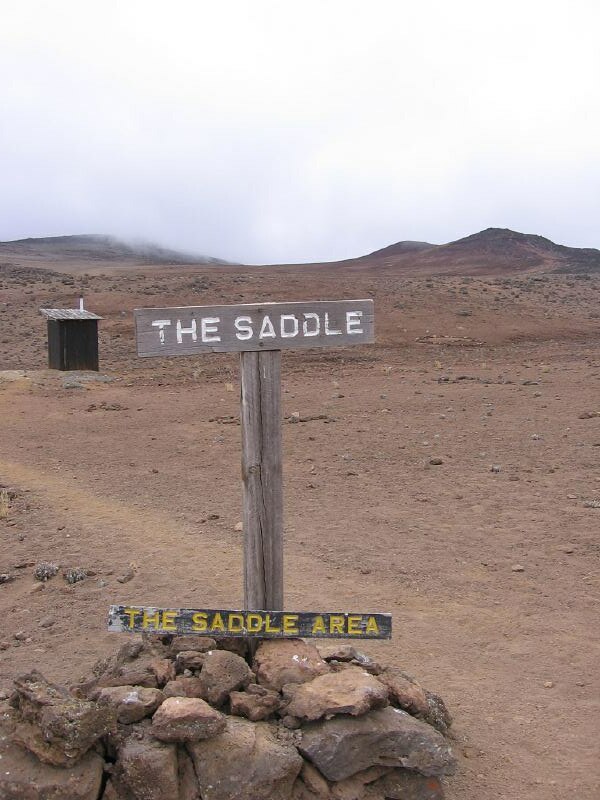The photograph captures a high-altitude desert landscape, characterized by sparse, rugged terrain and distant, cloud-covered hills. The scene is dominated by a vast expanse of dirt that stretches out to the horizon where the hills rise under a white, overcast sky. A wooden signpost, centered in the composition, features a wooden board with white lettering that reads "The Saddle." Off to the left of the signpost, a small, shack-like structure stands, possibly an outhouse or storehouse. In the foreground, a pile of rocks, about two feet high, supports a worn wooden sign with yellow text that reads "The Saddle Area," lying amongst the rubble. The overall sense of isolation is reinforced by the lack of vegetation, attributed to the high altitude of the location.